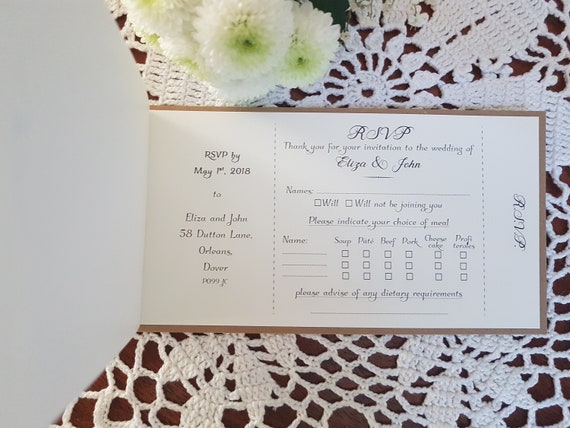The photograph showcases a wedding RSVP card set on an elegant, lacy table covering, often referred to as a doily, which rests upon a dark brown table. The RSVP, made of card stock featuring a brown border with a cream-colored interior, is positioned centrally within the frame. The text on the card gracefully thanks the recipient for their invitation to the wedding of Eliza and John, and instructs them to RSVP by May 1st, 2018. The card also provides dining options, including soup, pate, beef, pork, and cheesecake. Above the card, in the upper middle section of the image, a bouquet of white flowers adds a touch of natural beauty, although only the flower heads are visible. The scene is captured from a top-down perspective, emphasizing the intricate details and careful arrangement of each element.